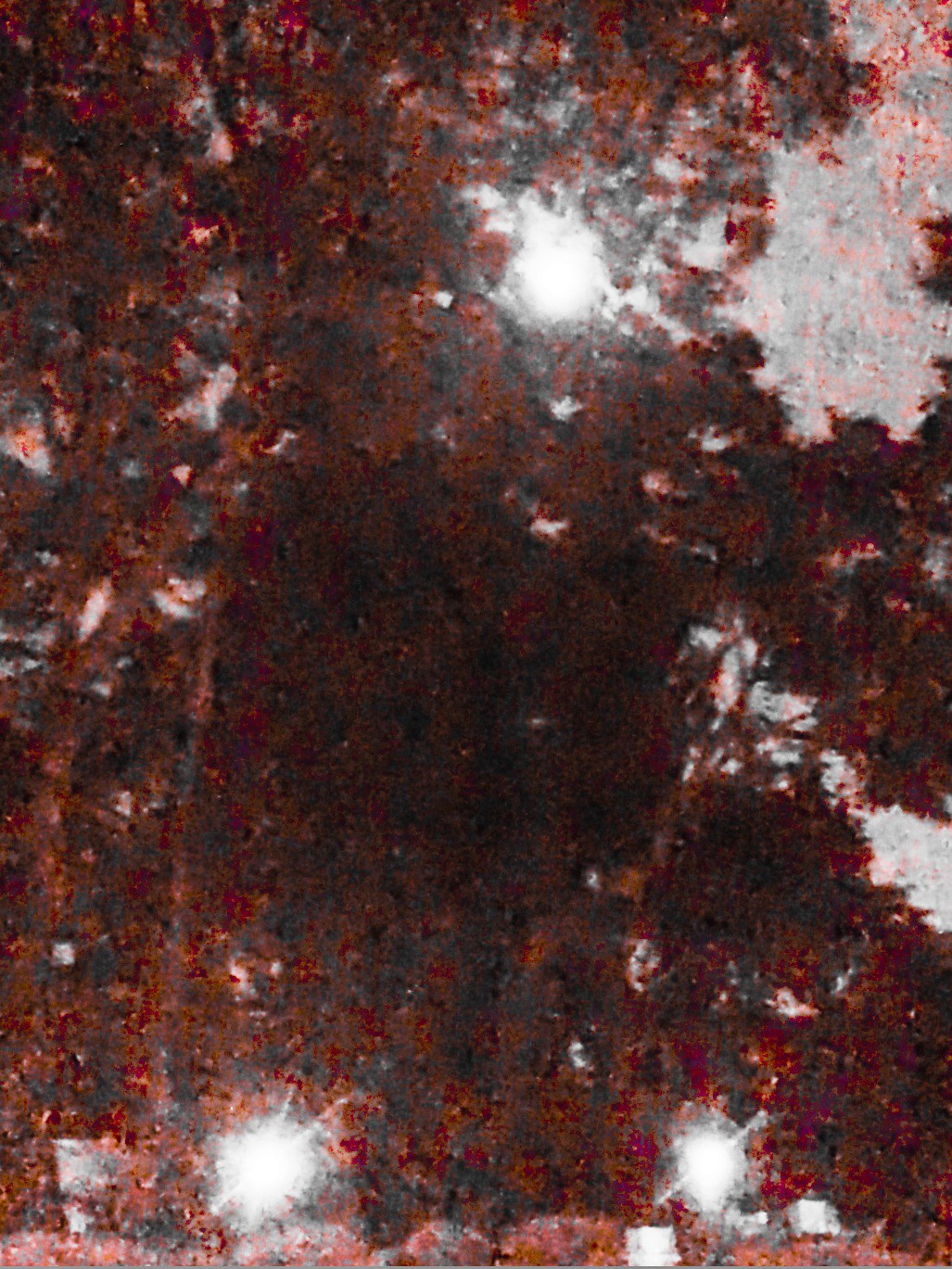The image appears to be a highly blurry, low-resolution photograph, likely taken outdoors, depicting a scene with trees. The overall coloring of the photograph is heavily tinted in shades of burgundy red and dark brown, which seems to distort the natural colors, lending the image an almost painting-like quality. The trees seem to be deciduous, as they have broad leaves that appear to have changed color, suggesting a fall setting. The composition features long, thin tree trunks ascending into the sky, with clusters of red and reddish-brown leaves scattered around. The branches and tree bark are outlined in dark brown or black, adding contrast and depth to the image.

There are sparse areas among the leaves, allowing sunlight to penetrate and create small circles of light, highlighted in white. This effect gives an impression of rays shining through the canopy. Notably, there are lighter patches towards the top and the top right of the image, where the light filters through the foliage. Additionally, the bottom left and bottom right areas also have hints of lightening, likely due to direct sunlight or intentional shading to emphasize these sections.

Furthermore, there's a visible bright ball of light at the top, possibly the sun, casting a glare that is further distorting the colors and adding to the pixelated appearance in certain areas, especially the top right corner. The left side of the image features elongated tree trunks reaching skyward, surrounded by a burst of red leaves. On the right, aside from the trees and leaves, there are glimpses of the sky peeking through the dense foliage. The ground below seems uneven, with some reddish stones and white flashing lights visible, adding a mystical touch to the entire scene.